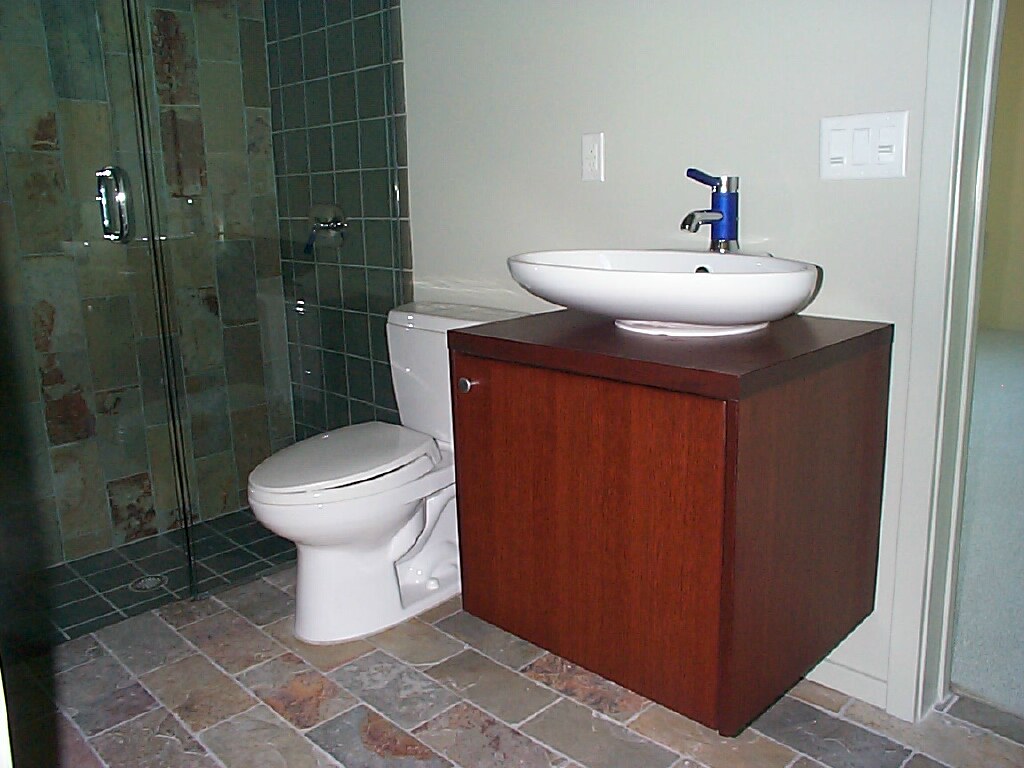This photograph depicts the interior of a pristine, brand new bathroom. The right side of the room features a white wall with white wooden molding. Mounted on this wall is a brown wooden square with another brown square attached on top. Below this setup, a white sink basin is installed, complemented by a modern, blue faucet extending from the wall. Above the faucet, two large white switches are mounted on a white plastic switch base, which can be pressed at the top or bottom.

To the left of the sink is a white porcelain toilet, set against a white wall. Dominating the left side of the photo is a two-door glass shower enclosure. The wall behind the shower features gray tiles, with an intricate design made from different shades of gray tiles on the right wall, mirroring the pattern on the bathroom floor. A partially open door is visible on the right side of the image, providing a glimpse into another room.